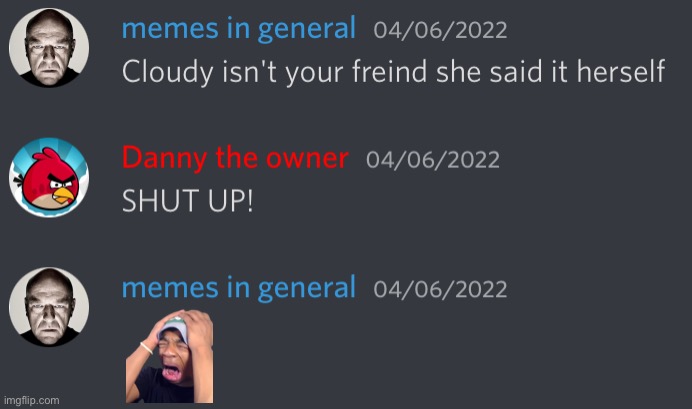A screenshot from a website, featuring a black background, is displayed in landscape mode with a small white text "imgflip.com" located in the very bottom left corner. The image shows a thread of three posts involving two distinct user profile pictures. The first and third posts, identified by a black and white photo of a bald man with a severe expression and bushy eyebrows, are from the user "memes in general." The second post comes from "Danny the owner," represented by the profile picture of the red bird from the Angry Birds franchise.

The thread begins with a post from "memes in general," dated 04-06-2022, written in blue text with the message, “cloudy isn't your friend she said it herself," with the word "friend" misspelled as "freind." 

Danny the owner replies on the same date in bold red text, shouting in all caps, "SHUT UP!"

Following this, "memes in general" responds again on 04-06-2022 by posting a photo of an African American man with his hands clasped over his ball cap, displaying an expression of either crying or disappointment.